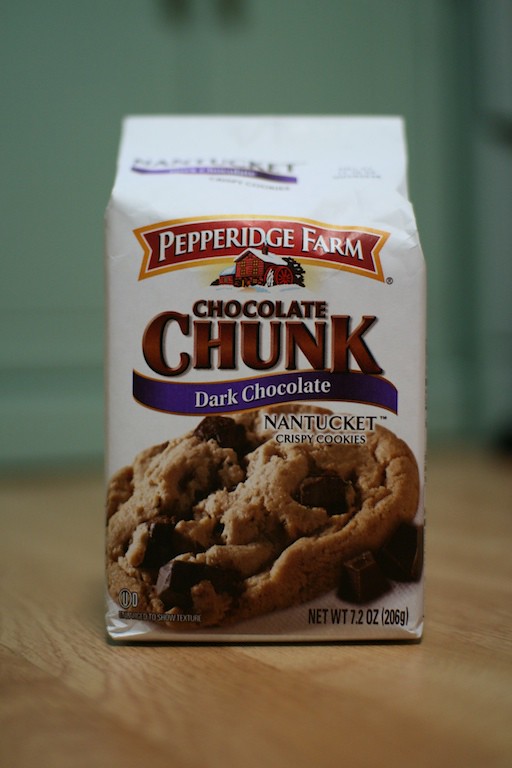Displayed on a wooden laminated table, the photo features a package of Pepperidge Farm Chocolate Chunk Crispy Cookies. The backdrop, a slightly out-of-focus peppermint green wall, adds a soft contrast to the scene. The cookie packaging is predominantly white and has a gathered top, reminiscent of a non-transparent cereal packet liner. Adorned with a brown banner outlined in gold, the Pepperidge Farm logo is prominent. A charming illustration of a house, made to look like chocolate, adds a touch of whimsy, while a tantalizing image of a gooey, delicious cookie is prominently displayed, tempting the viewer. The packaging clearly states the net weight: 7.2 oz (206g).